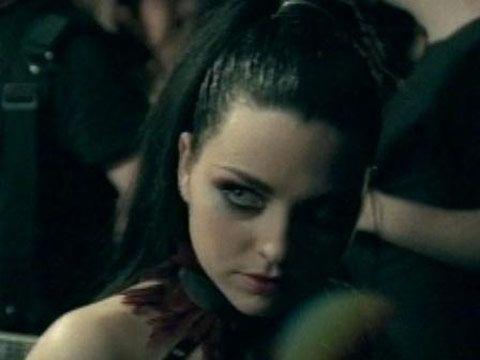This grainy and low-resolution image features a white woman, possibly the singer Amy Lee from Evanescence, exuding a gothic presence. Her black hair is pulled back into a long ponytail cascading down her back, with a section pulled out of her eyes. She sports heavy, dark eyeshadow that accentuates her light, possibly blue, eyes, and she complements this look with dark red lipstick. Her expression is one of anger or intense emotion, and she is casting a side-eyed look towards the left. Around her neck is a choker adorned with dark red feathers that partially covers her bare shoulder. The right side of her face is shrouded in shadow. In the blurred background, there are at least two indistinct figures, one on the left wearing a black outfit with only an elbow visible, and another on the right with a black outfit and an arm faintly discernible. The overall setting appears dark, contributing to the moody atmosphere of the image.